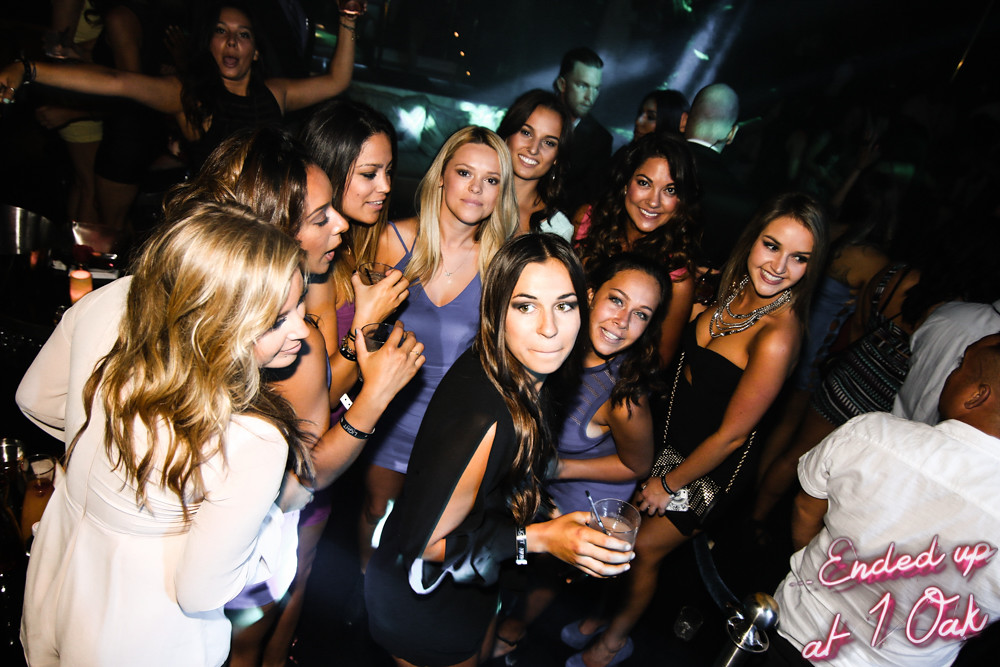This color photograph captures an energized moment inside a dimly lit nightclub, prominently featuring a group of about ten young women in their 20s or 30s. The scene is illuminated perfectly to spotlight the women amid a dark backdrop, with the words "Ended up at One Oak" displayed in white and pink letters in the bottom corner. Dressed to impress in short, stylish dresses ranging from black to purple, these women exude glamour with their makeup carefully done, long hair cascading down, and adorned with lots of jewelry. They each hold small drinks and little purses, showcasing the typical club attire. The photograph is taken from a slightly elevated angle, contributing to the dynamic yet intimate feel as the women stand close together, smiling, posing, and engaging with one another. The viewer’s attention is drawn to their expressions and interactions, framed by a subtle presence of shadowy figures in the periphery, heightening the sense of a lively, exclusive night out.